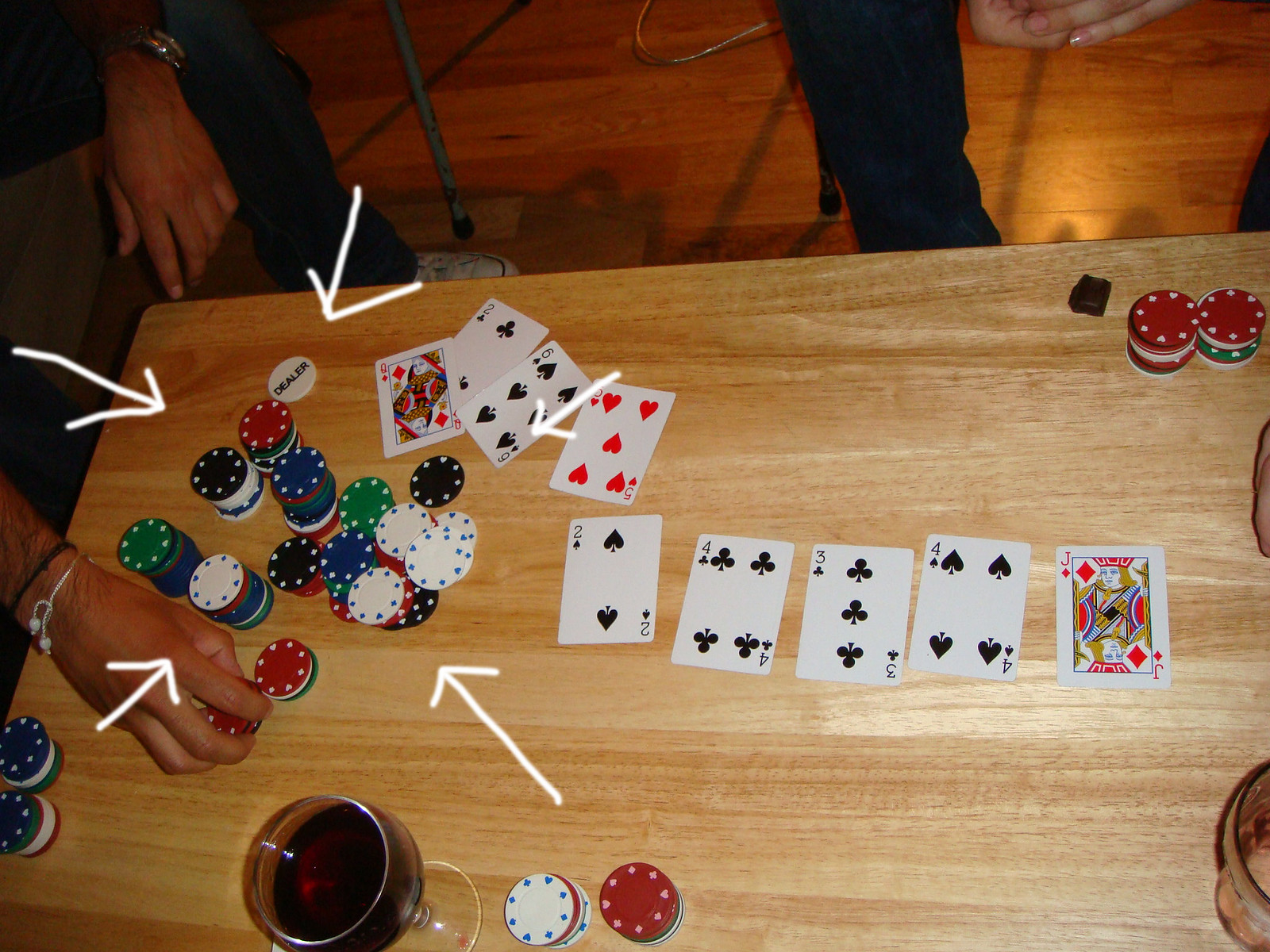In this image, we get an overhead view of an intense poker game in progress. At the very bottom of the scene, there's a half-filled wine glass containing a dark red to almost black wine. The poker game is set on a light brown wooden table, which lends a warm and rustic atmosphere to the scene. 

On the bottom left corner, there are two neat stacks of poker chips, comprising white, green, red, and blue chips, with blue chips on top. Directly to the right of these stacks is the wine glass, and then another pair of chip stacks follows, featuring a white chip on the left stack and a red chip on the right stack.

To the left side of the table, we see five arrows that point towards a series of poker chips. Above these chips, four poker cards are laid out: the Queen of Diamonds, the Two of Clubs, the Six of Spades, and the Five of Hearts.

Below these cards, five more cards are displayed: the Two of Clubs, the Four of Clubs, the Three of Clubs, the Four of Spades, and the Jack of Diamonds. Towards the top right of these cards are two additional stacks of poker chips, both having red chips on top.

In the background, a hand is partially visible, with another hand on the left side gripping a stack of poker chips. The backdrop includes an orangish-brown wooden wall and a blue towel hanging, adding to the cozy yet competitive ambiance of the poker game.